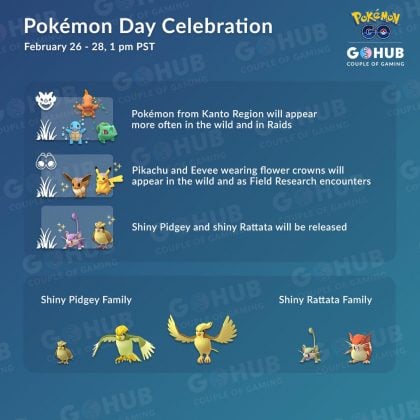This detailed caption better describes the content and visual elements of the image:

---

This image is an information page from GoHub, dedicated to Pokémon Go. In the upper right-hand corner, the word "Pokémon" is displayed in a familiar yellow font, followed by the word "Go" in a bold blue font. Adjacent to this, the GoHub logo appears, featuring "GoHub" in white text, with the 'O' stylized to resemble a small globe.

On the left side of the page, large text announces a "Pokémon Day Celebration" taking place from February 26 to 28, starting at 1 p.m. Pacific Standard Time. The background is a deep blue, subtly patterned with faint, diagonal imprints of the words "GoHub" and "Couple of Gaming," running upwards towards the right across the screen.

Three major announcements are highlighted on the page:
1. Pokémon from the Kanto region will appear more frequently in the wild and in raids. This is illustrated with images of various Pokémon.
2. Pikachu and Eevee, both adorned with flower crowns, will appear in the wild and as field research encounters. Icons of the Pokémon next to this announcement include binoculars, indicating their availability through field research.
3. Shiny Pidgey and Shiny Rattata will be newly released, accompanied by images of these Pokémon.

At the bottom of the page:
- The "Shiny Pidgey Family," accompanied by illustrations of three shiny Pokémon.
- The "Shiny Rattata Family," depicted with images of two shiny Pokémon.